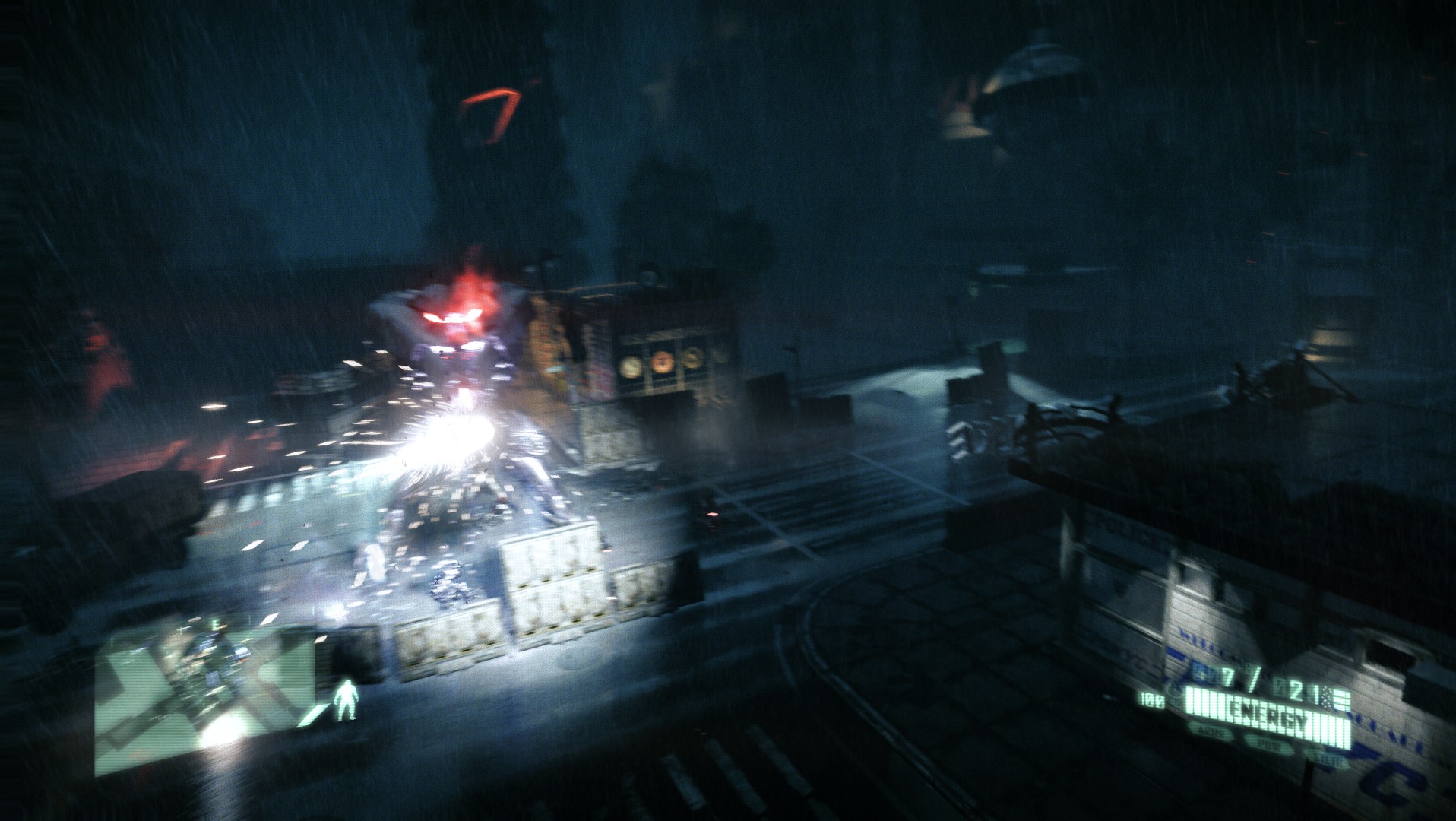This image is a still from a video game set in a detailed 3D environment, depicting a futuristic cityscape at night. The scene is viewed from an elevated perspective, showing a complex maze of illuminated roads and buildings below a dark, rain-soaked sky. On the left side of the image, a towering robot with vivid red lights emanating from its head area stands ominously, surrounded by bright white sparks. The ground near the robot features a partially legible sign, adding to the mystery of the setting. The right side of the image is illuminated by lights from a notable structure, while in the background, the silhouettes of more buildings fade into the night. The bottom left corner of the screen displays a mini-map, highlighted by a small white silhouette indicating the player's position. In the bottom right corner, there is an energy bar, reading "Energy: 7/21," suggesting resource management as a gameplay element.